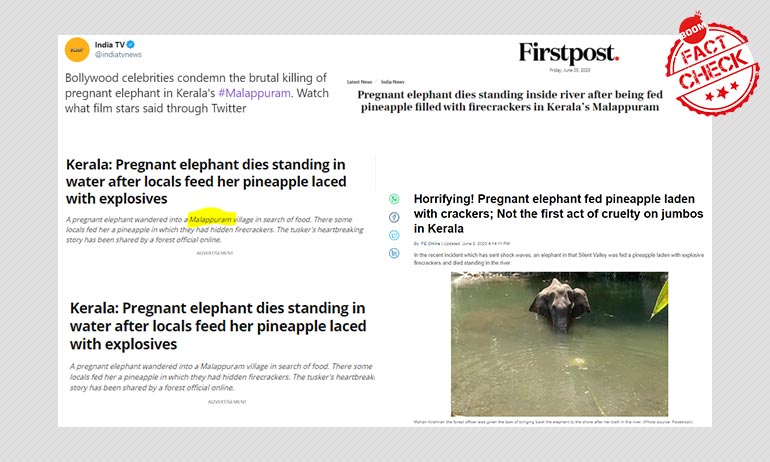The image captures a webpage from India Times, reporting on Bollywood celebrities' condemnation of a tragic incident in Kerala's Malappuram. The headline highlights the brutal killing of a pregnant elephant, which succumbed to injuries after being fed a pineapple filled with firecrackers. The poignant photograph shows the elephant standing in a river, where she ultimately died. This horrifying act has sparked outrage, making headlines as not the first instance of cruelty towards elephants in Kerala. The heart-wrenching story is further amplified by the reactions of fame stars on Twitter, expressing their grief and demanding justice for the innocent creature.